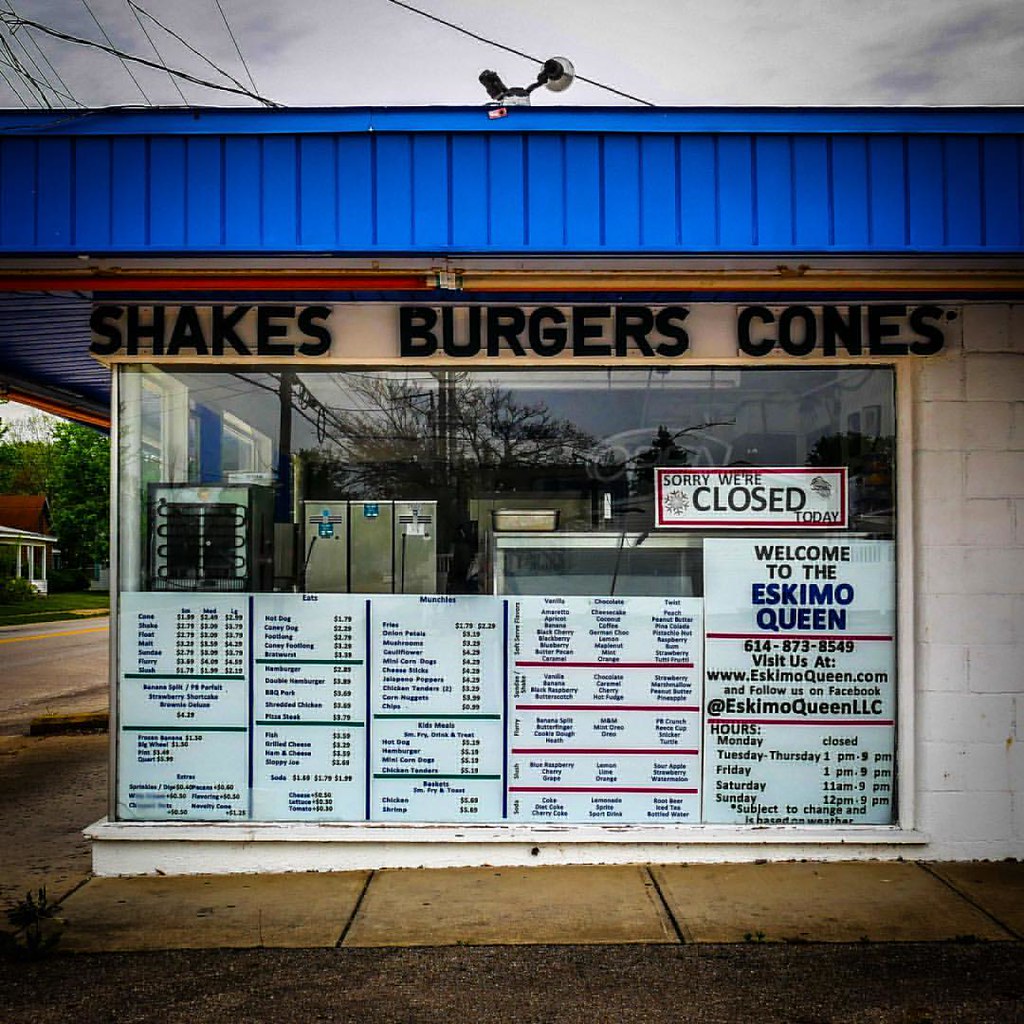The photo showcases the exterior of a charming, old-style restaurant named "Eskimo Queen." Above its large blue roof, prominently displayed in black lettering, are the words "Shakes, Burgers, Cones." A red-outlined box in the window bears a sign that reads, "Sorry, we're closed today," indicating the photo was taken on a Monday, their designated closed day. Detailed operational hours are listed: Tuesday to Thursday from 1 p.m. to 9 p.m., Friday from 1 p.m. to 9 p.m., Saturday from 11 a.m. to 9 p.m., and Sunday from 12 p.m. to 9 p.m. The restaurant's contact information includes a phone number, 614-873-8549, a website, www.eskimoqueen.com, and a call to follow them on Facebook at Eskimo Queen LLC. While the handwritten menu across the lower part of the building’s wall is somewhat difficult to read from a distance, it mentions a variety of offerings such as shakes, ice cream, burgers, sodas, kids meals, and basket options like chicken, shrimp, and more, contributing to its nostalgic diner appeal.